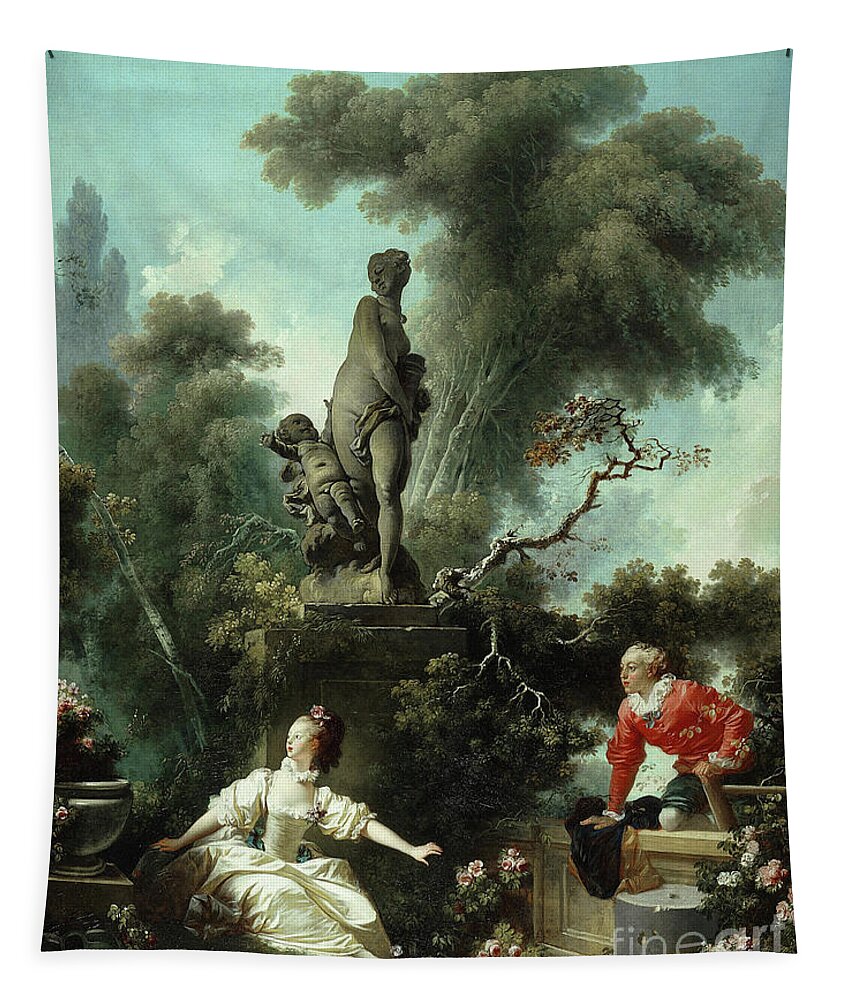The image depicts an antique Victorian-era oil painting, set on a tapestry-like canvas. At the center, a Roman-style statue of a woman stands elevated on a platform, a child resting against her hip without her holding it. The background features green trees and a sky shrouded in dull colors, creating a slightly smoky or unclear atmosphere. In the foreground, a young girl in a white silk dress, with puffy sleeves and a high collar, is positioned at the base of the statue, her hair adorned with a rose-colored flower. She appears startled, looking back over her shoulder as if fleeing from something. To her right, a boy in a red shirt with a white collar kneels, his right hand gripping his black coat, similarly gazing in the same direction with a surprised expression. Roses surround the scene, adding vibrant details to the otherwise muted background.